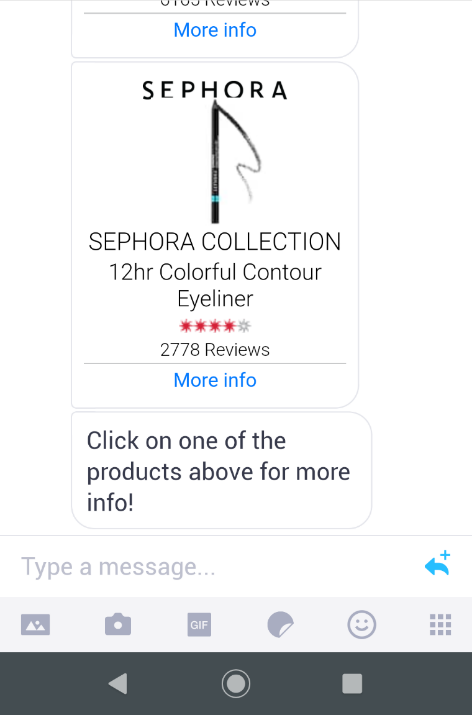A cellphone screen capture displays a Sephora product page for colorful contour eyeliner. The top portion of the image shows a partial view of a different product listing with only the "More Info" link visible in blue. In the center of the image, the Sephora logo is prominently featured alongside a depiction of the eyeliner pencil. A swatch of the eyeliner is shown below, illustrating a vibrant squiggly line drawn in a sample color. The product is identified as "Sephora Collection 12-Hour Colorful Contour Eyeliner" and is rated four out of five stars, based on 2,778 customer reviews. Beneath this information is another "More Info" link in blue. The screen also includes a navigation prompt to "Click on one of the products above for more information," along with a text entry field and a blue arrow icon next to a plus sign for additional actions.